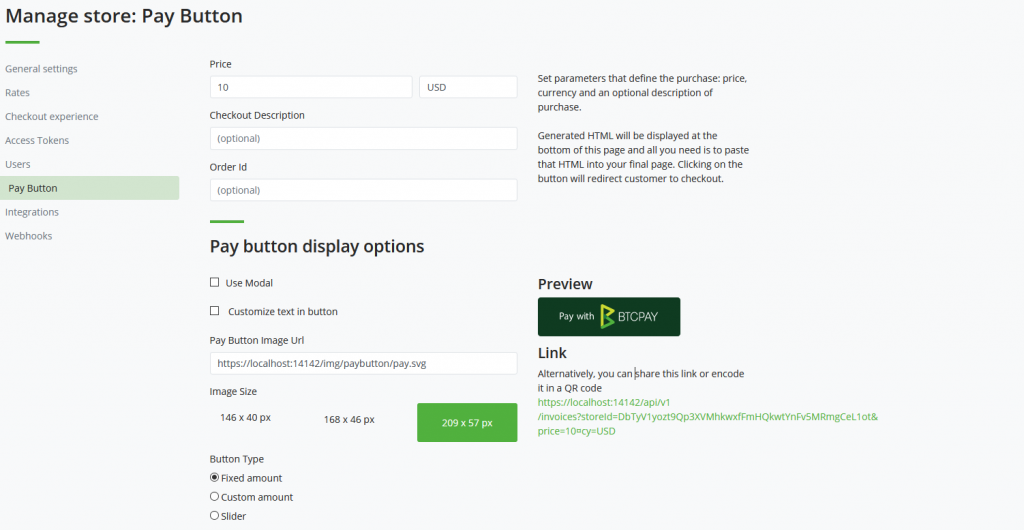The image depicts a user interface taken from a website. In the top left corner, there is bold text reading "ManageStore.payButton". Below it, a green line separates it from a list of options: General Settings, Rates, Checkout Experience, Access Tokens, Users. The currently selected option, "PayButton", is highlighted in green and bold.

Directly underneath this, the words "Integrations" and "Webhooks" are displayed in regular gray text. The main section of the interface seems to focus on the settings for a feature called "PayButton". At the top center of this section, a price field displays "10 USD". The fields for Checkout Description and Order ID are both marked as optional.

Highlighted in bold, the "PayButton display options" section offers two checkboxes labeled "Use Module Model" and "Customize Text and Button"; these are currently unchecked. Another field labeled "PayButton Image URL" contains a web address, and below, there are three image size options. The selected size is highlighted in green: 209 by 57 pixels.

To the right, the button type is specified as "fixed amount". The rightmost column provides a detailed explanation, stating: "You can set parameters that define the purchase price, currency, and an optional description of purchase. Generated HTML will be displayed at the bottom of this page, and all you need to do is paste that HTML into your final page. Clicking on the button will redirect a customer to checkout."

A preview area features a banner that reads "PayWithBit BTC Pay", with an accompanying link. An alternative option is offered for sharing this link or encoding it into a QR code, highlighted by a green clickable text link.